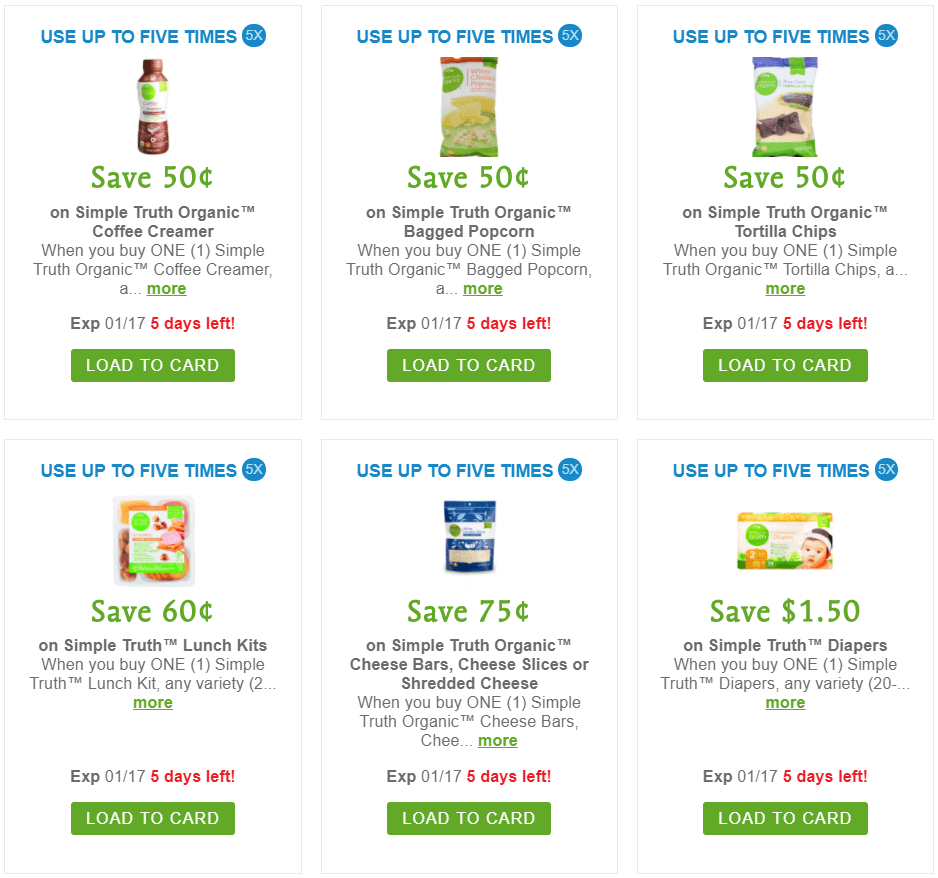This image is a screenshot taken from an e-commerce grocery site, showcasing a variety of digital coupons. There are six coupon options displayed in a grid format, three columns wide and two rows deep. Each coupon features bold blue text at the top and a blue circle with "5X" indicating the number of times the coupon can be used. Below this, green "Load to Cart" buttons are present for each coupon. Additionally, the phrase "Expires in 1/17" is shown along with a red notice indicating "5 days left."

The coupons offer the following discounts:

1. **Simple Truth Organic Coffee Creamer**: Save $0.50. The coupon displays an image of a bottle of coffee creamer.
2. **Simple Truth Organic Popcorn**: Save $0.50. An image of a bag of organic popcorn is shown.
3. **Simple Truth Organic Tortilla Chips**: Save $0.50. This option features a picture of blue tortilla chips.

On the second row:

4. **Simple Truth Lunch Kits**: Save $0.60.
5. **Simple Truth Organic Cheese**: Save $0.75. This includes cheese bars, cheese slices, or shredded cheese in a blue bag.
6. **Generic Diapers**: Save $1.50.

In each case, the discount amount is prominently displayed in green text, while additional details and qualifiers, such as "when you buy one," are in darker gray text. The layout and details suggest that this screenshot could be a mock-up for user interface testing or promotional purposes.